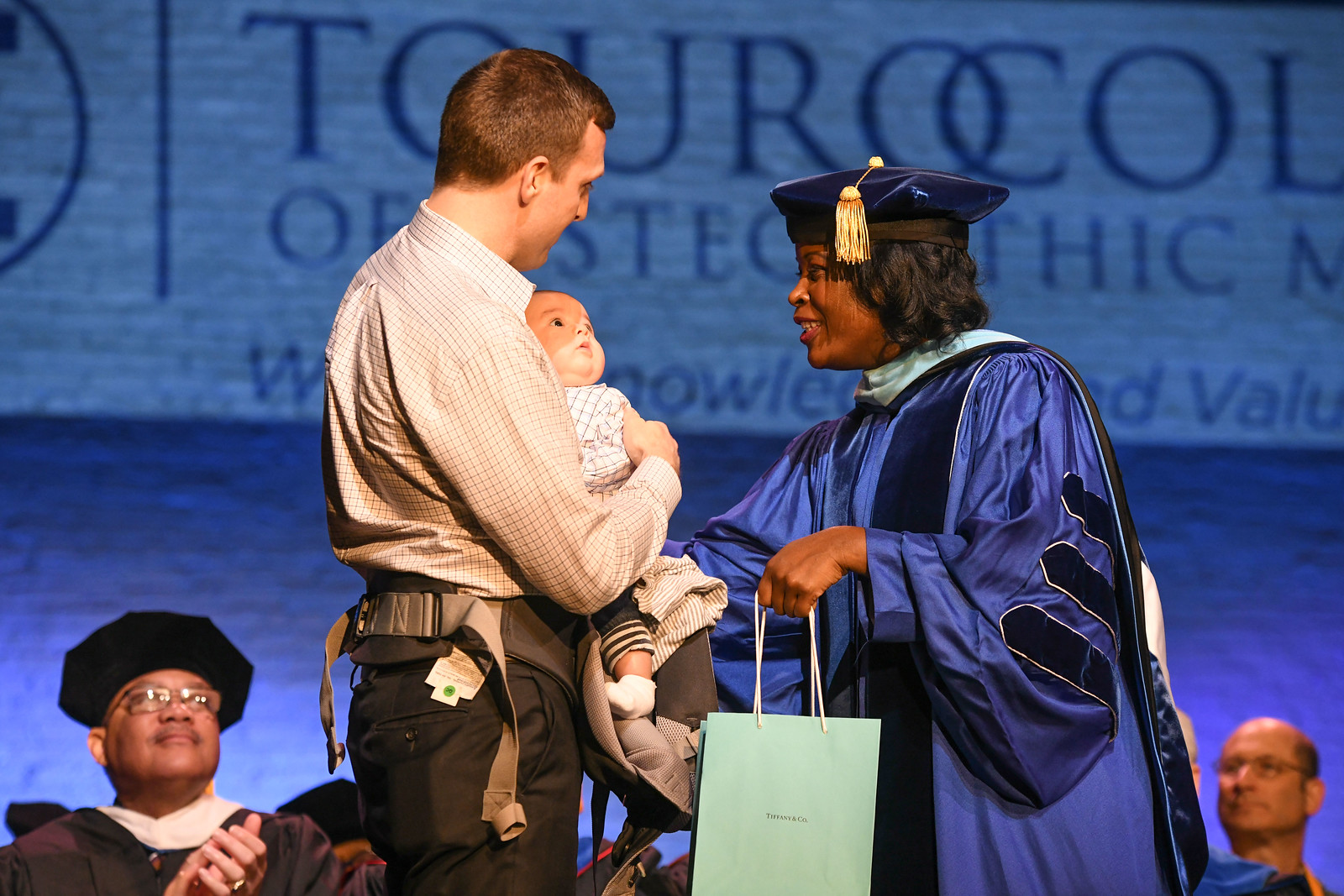The image captures a vibrant graduation ceremony with a blue-themed backdrop featuring a partially obscured sign that reads "Touro College" in dark blue lettering on a light blue background. Central in the scene is a jubilant African American woman dressed in a blue graduation gown and cap adorned with a gold tassel. She stands to the right of a light-skinned man with short brown hair, wearing a light button-up shirt and dark pants, who is holding a baby dressed in white socks and blue jeans, strapped securely to his chest. The woman is holding a light blue-green tote bag. Flanking the duo is an African American man, seated and clapping, adorned in a cap and gown, and to the far right, the head of another man with glasses is partially visible.